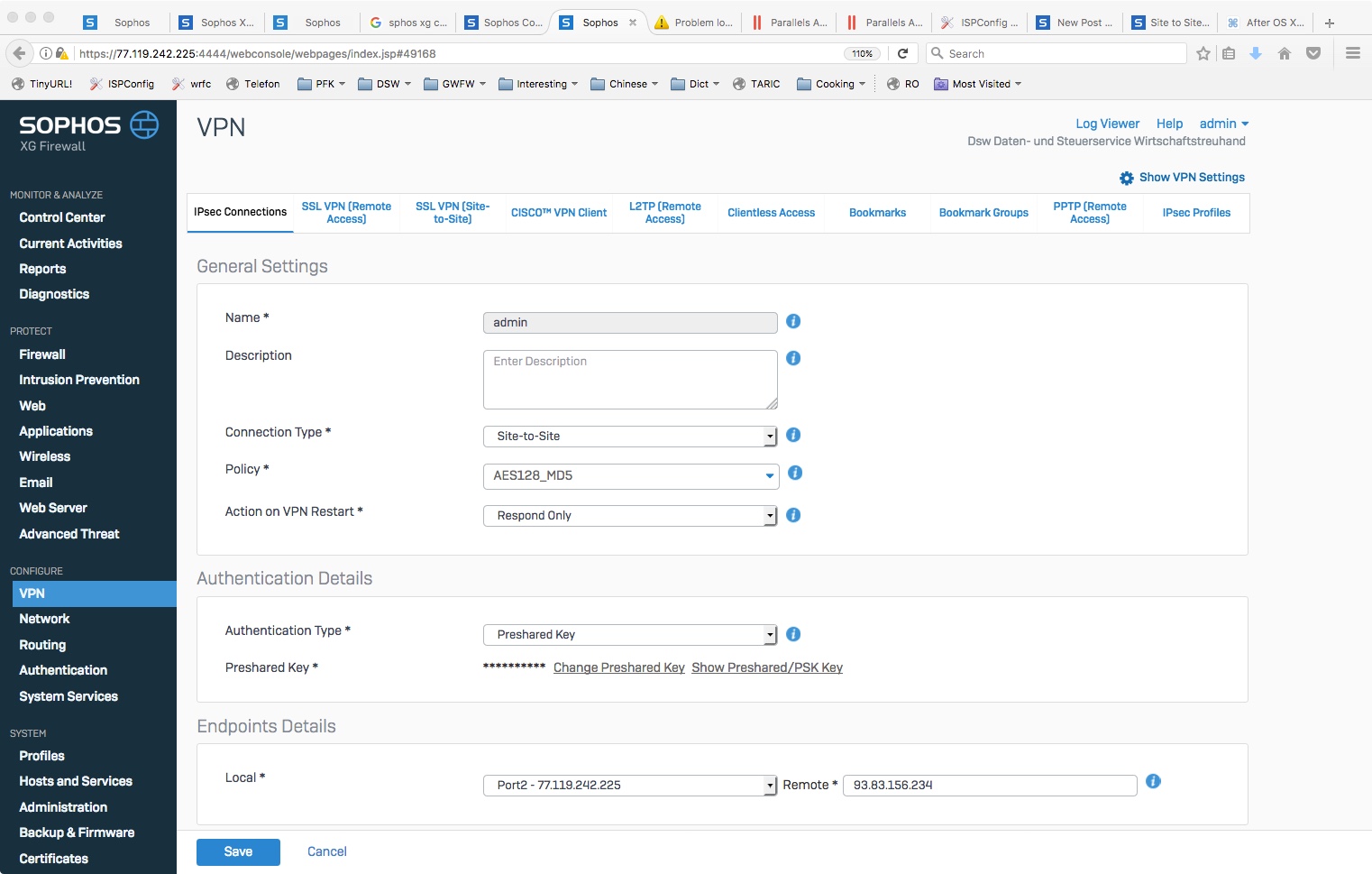A screenshot of a Google Chrome browser displaying multiple open tabs and a cluttered bookmark bar. The top section of the browser includes a header with options such as "VPN Log Viewer," "Help," "Admin," "Show VPN Settings," "VPN Client," "Bookmarks," and "Bookmark Groups." The image is somewhat blurry, making the text difficult to read. Below the header is a section labeled "Name" with a corresponding text box. There is also a field labeled "Admin Description" with another text box prompting to "Enter Description." Other visible fields include "Connection Type" set to "Site-to-Site" and "Policy," though the details are unclear due to the blurriness. There is an action option labeled "Action on VPN Restart" with "Respond Only" as its setting. The "Authentication Details" section has fields for "Authentication Type," "Key Change Interval," and a checkbox for "Show Settings." Additionally, there is a "Local Authentication" section visible. The overall interface appears to pertain to VPN configuration settings, though specific details are hard to discern.